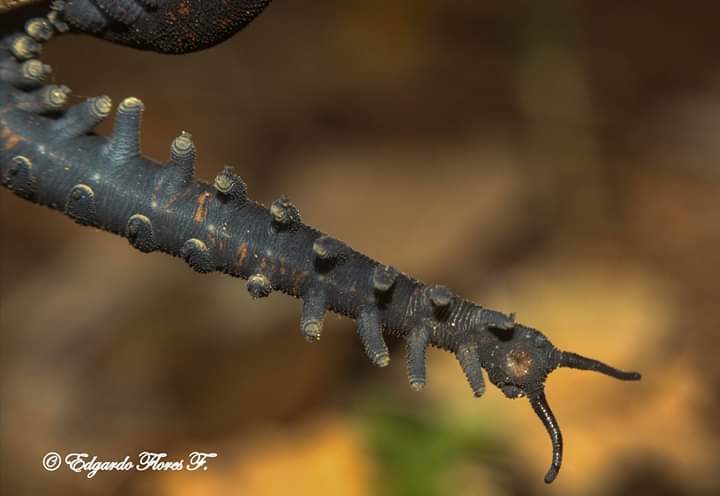This detailed nature photograph, captured and copyrighted by Edgardo Flores F., showcases a close-up of a presumably caterpillar-like creature. The image highlights the front part of the long, tubular insect, positioned diagonally from the top left to the center of the frame. The caterpillar appears to be coiled, with a segmented or ridged body, suggestive of its climbing abilities. Prominently visible are its many small, rounded legs, each jutting out in various directions and resembling corrugated metal. Its underside and feet are distinctly detailed. Two thick, large antennae curl gracefully, mirroring the curvature of its legs. The face of the caterpillar appears to have what might be eyes and a small, brownish mouth opening, though these features are somewhat ambiguous. The backdrop of the image is heavily blurred, composed of basic brown and orange hues, leaving the focus purely on the insect and providing no clear sense of its actual size or environment.